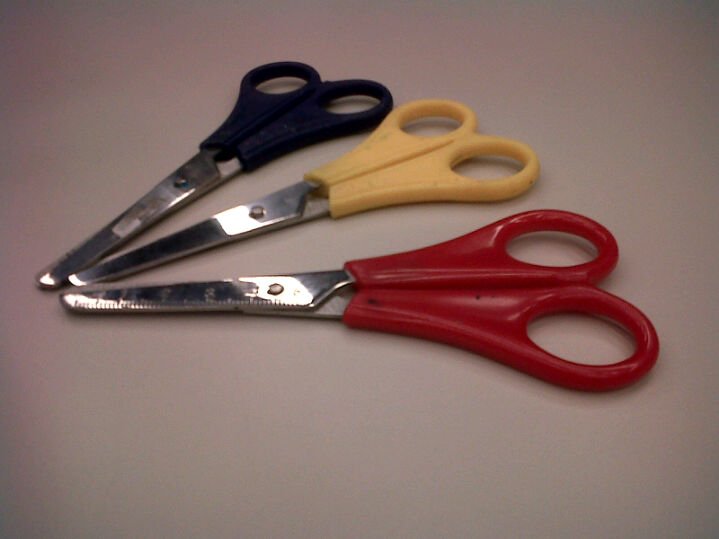This photograph features three pairs of child safety scissors arranged on a dimly lit white or light brown background with a vignette effect. The background is slightly wider than it is tall. The scissors are positioned in a curved arc formation, with their closed blades converging towards a mid-height point on the left side of the image, as if pointing at 9 o'clock, 8 o'clock, and 7 o'clock from bottom to top respectively. The handles, made of thin plastic, are distinctly colored in red for the bottom pair, yellow for the middle pair, and dark blue (mistaken for black or silver in different accounts) for the top pair. The rounded ends of the scissors indicate they are designed for children, and there's a noticeable glare on the silver blades, highlighting their metallic finish. The overall composition is simple, emphasizing the minimalist arrangement and child-friendly design of the scissors.